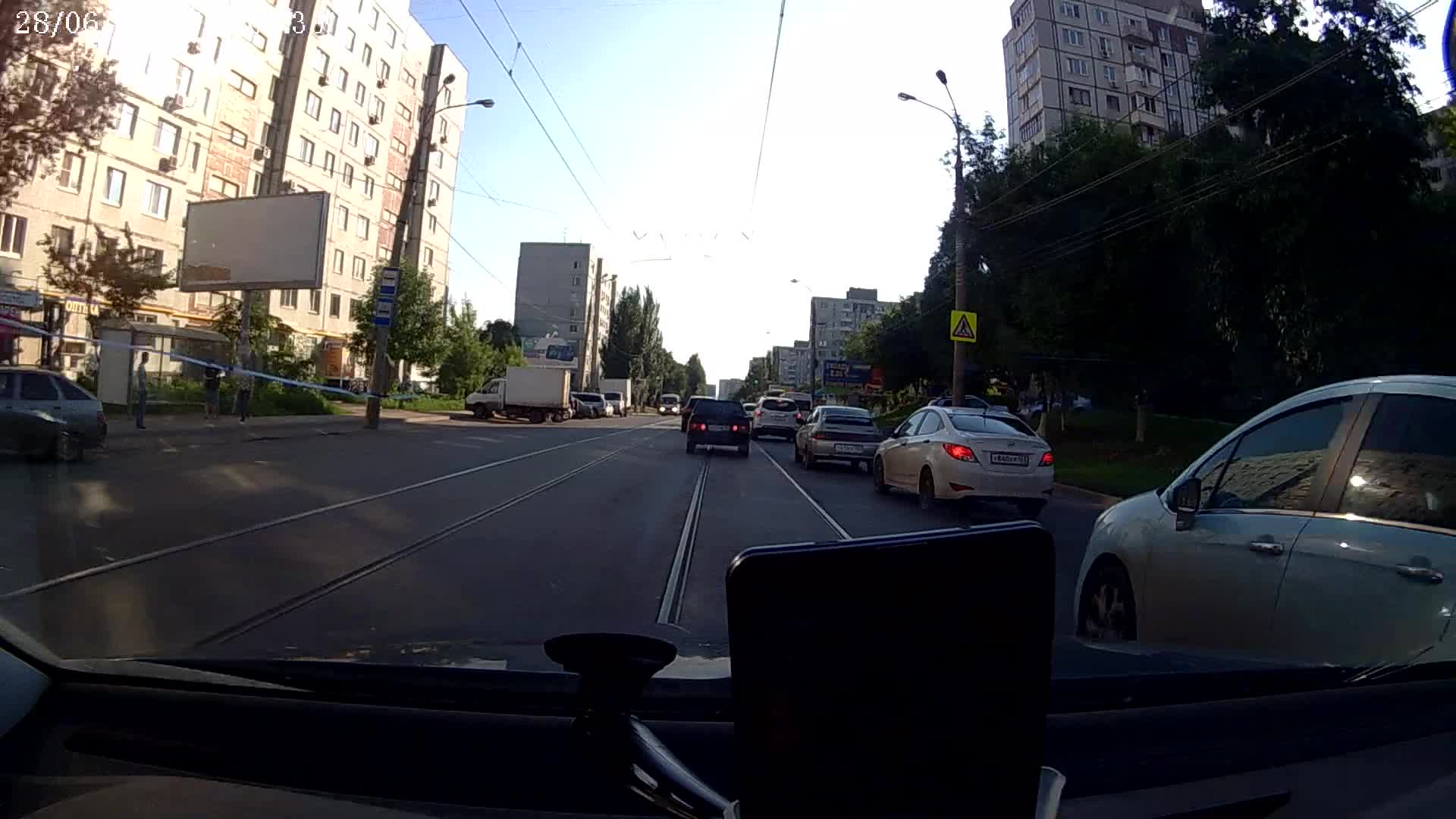This photograph, taken from inside a vehicle through what appears to be a wide-angle fisheye lens, showcases a busy urban street scene. In the bottom section of the image, the dark dashboard is visible, featuring a mounted cell phone or GPS unit slightly to the right. The shot looks straight down the road through the front windshield, with a teal or blue car positioned beside the vehicle, its rear driver’s side door in view. In front of this car is a white vehicle with its red brake lights illuminated. Multiple cars are seen ahead, suggesting the vehicles are stopped, possibly at an intersection.

On the sides of the street are tall buildings stretching out of frame. To the left, there's a large multi-story building, possibly an apartment or hotel, characterized by a flat front with numerous windows set into a brick facade. The structure extends beyond the top edge of the frame, indicating its substantial height. Similarly tall buildings are situated on the right, accompanied by trees in the foreground and light posts lining the street. Electrical wires crisscross above the road.

In the far background, the scene is set against a daytime sky, though the brightness causes a blown-out white area in the center, white-washing some details. Additionally, in the distant background on the opposite lane, a bus or truck is visible, indicating ongoing traffic approaching from afar. Overall, the image captures a dynamic street view with an array of urban elements.